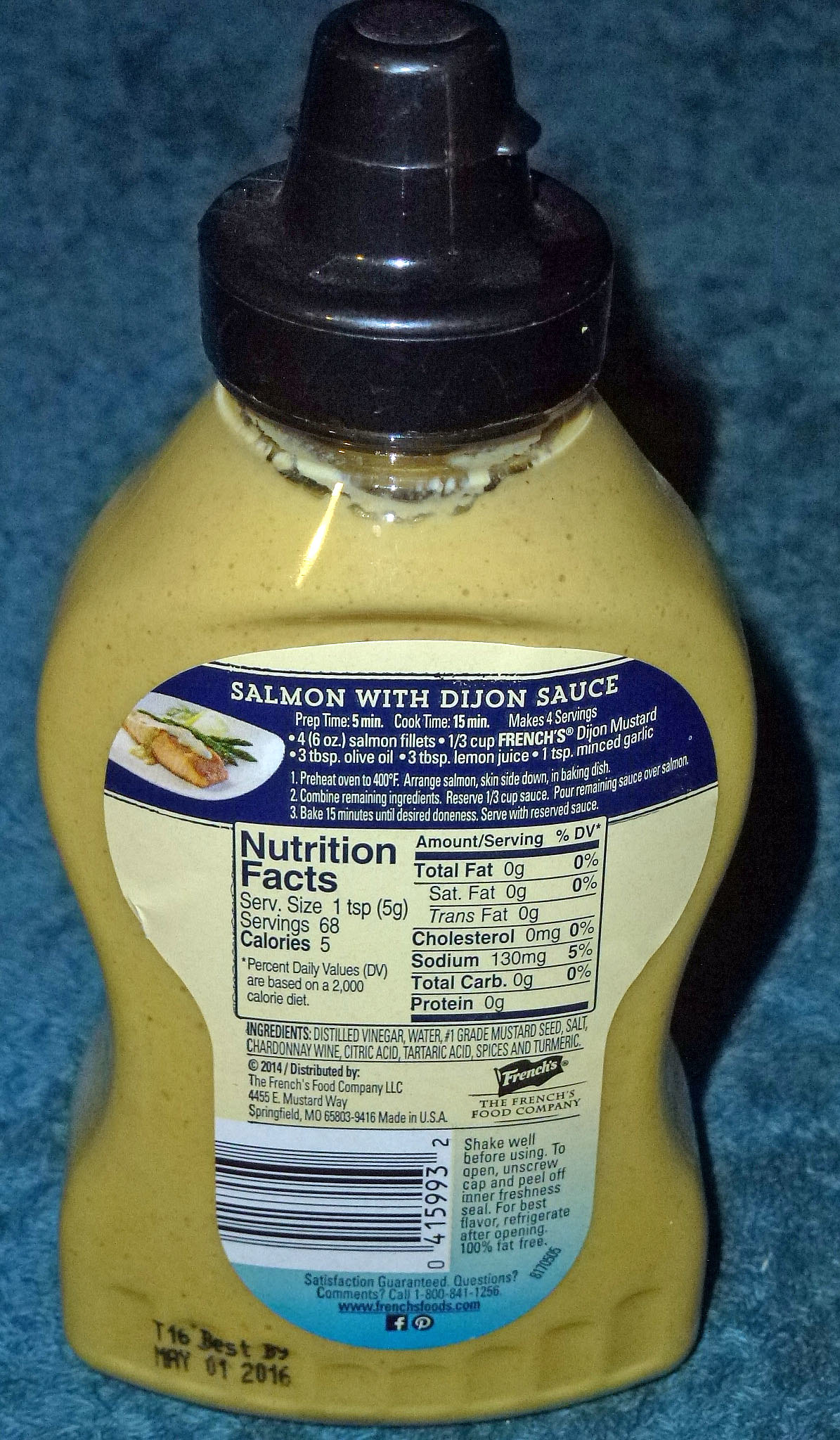The photograph in front of me is a colorful, portrait-oriented image. Dominating the foreground is a bottle of Dijon mustard, turned so that its back label faces the viewer. The mustard bottle rests on a medium blue, carpet-like or fabric surface. The lid of the mustard container is dark blue, featuring a pourable spout. The mustard inside is a pale golden yellow, almost light golden brown.

The white label on the back of the bottle is predominantly decorated with a blue banner that highlights a recipe for salmon with Dijon sauce. An illustrated plate on the label showcases a piece of pinkish salmon accompanied by asparagus. Below the recipe, nutritional facts are listed though somewhat blurry; it seems to indicate that the bottle contains approximately 60 servings with 5 calories per serving. At the very bottom of the label, in black lettering, is a "Best By" date of May 1, 2016.